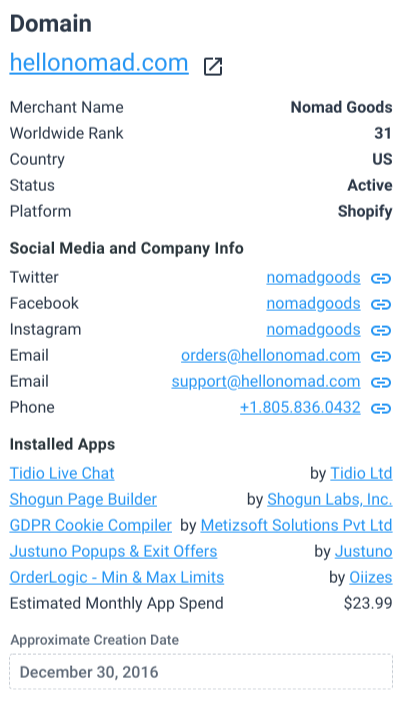The image depicts a domain page overview focusing on the domain "hellonomad.com," indicated prominently at the top of a white background filled with various pieces of information. The domain belongs to "Nomad Goods," a merchant with a worldwide rank of 30,731. The company is based in the US, has an active status, and operates on the Shopify platform.

Detailed information on social media and contact details include:
- Twitter: Nomad Goods
- Facebook: Nomad Goods
- Instagram: Nomad Goods
- Email for orders: orders@hellonomad.com
- Support email: support@hellonomad.com
- Phone number: +1-805-836-0432

Additionally, the image displays a list of installed applications:
- TDO Live Chat by TDO LTD
- Shogun Page Builder by Shogun Labs Inc.
- GDPR Cookie Complier by Medsoft Solutions PBT LTD
- Jasuno Pop-Ups and Exit Offers by Jasuno
- Order Logic Min and Max Limits by All Ease

The estimated monthly ad spend is noted as $23.99, and the approximate creation date of the domain is provided as December 30, 2016.